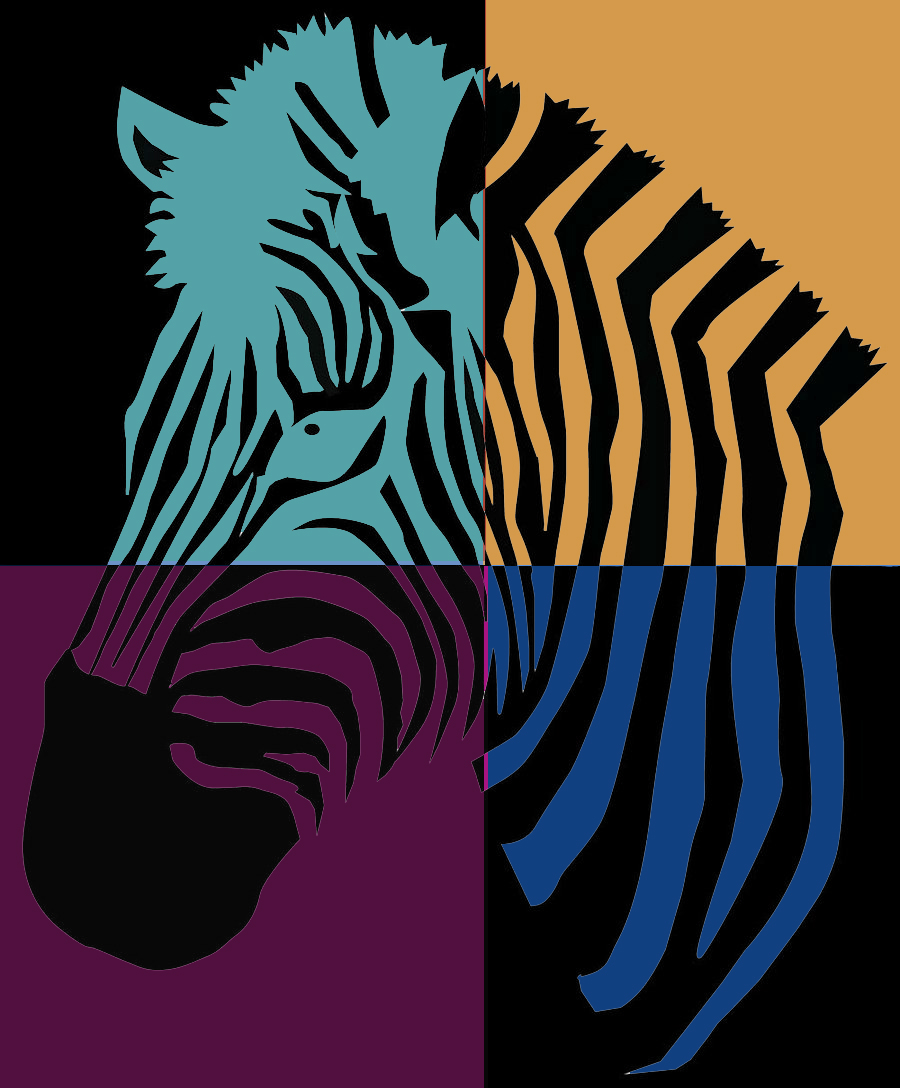This digital artwork features a stylized, black and white side view of a zebra, divided into four distinct rectangular sections, each uniquely colored. The image has a clip art or linoleum cut aesthetic, akin to a stamp, showcasing only the zebra's striped fur. The upper left quadrant displays a black background with the zebra rendered in teal. The upper right section contrasts with an orange background and traditional black stripes on the zebra. The lower left portion features a plum backdrop with the zebra's stripes also in black, while the lower right corner returns to a black background but with the zebra's stripes in blue. Through these four quadrants, the piece maintains the same image of the zebra, yet each section's distinct coloration provides a dynamic, abstract presentation. The zebra retains an oval-shaped eye filled in black, creating a lively and colorful representation of this majestic animal.